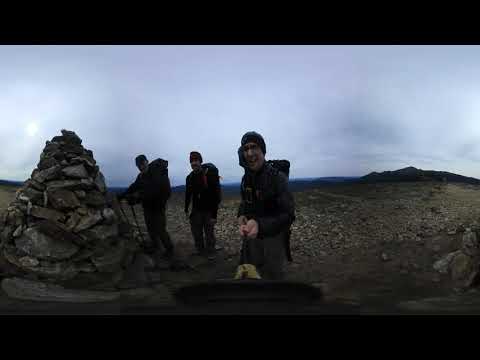In the photograph, a group of three men, all bundled in warm black outfits and hats, are taking a selfie with a black selfie stick. The man in the forefront, who is smiling and holding the stick, is dressed in a black long-sleeve shirt, brownish pants, and has a large backpack on his back. This rocky and desolate landscape appears devoid of plant life, with rough terrain underfoot and a notable cairn to the left of the group. The sky overhead is overcast, casting a dull grayish hue across the scene, while the distant backdrop reveals the silhouettes of mountains or large hills. The overall atmosphere is one of cold and stark wilderness, accentuated by the men's warm clothing and the absence of greenery.